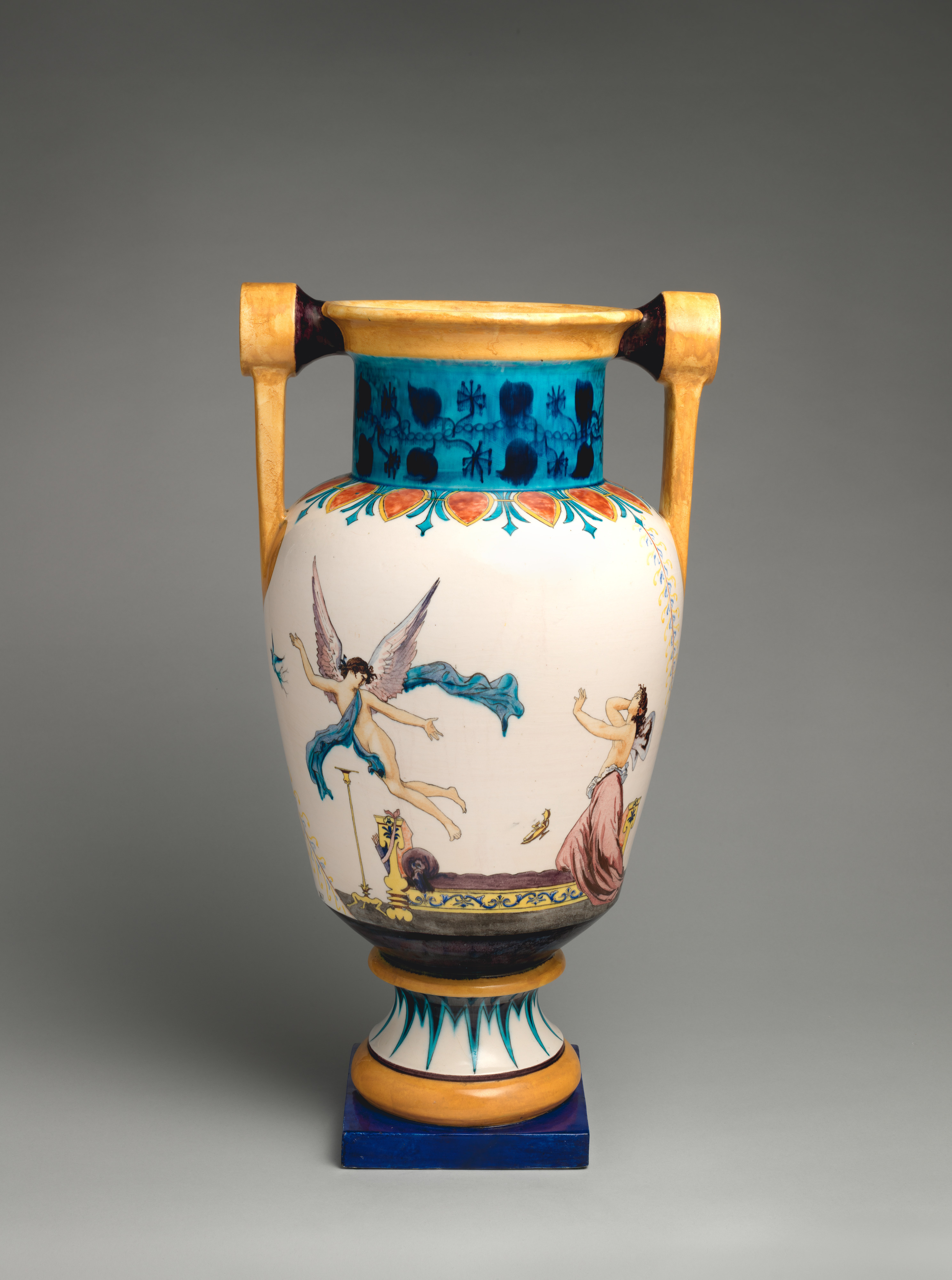The image depicts an intricate vase set against a plain gray background, possibly intended for a professional photograph. The vase stands on a solid blue square base, resembling a thin brown wafer in shape. Its narrow bottom flares into a wider main body before tapering again at the neck, which features blue abstract designs. The vase has two wooden-looking handles on each side. The neck is brown along the rim and blue above it with abstract motifs.

The main body of the vase displays a classical scene reminiscent of Roman art. A male angel with white wings, naked except for a flowing blue fabric covering his chest and genitals, is depicted flying above. To his right, a topless woman, partially clothed in a pinkish dress pulled down to her waist, is shown in a pose of distress or longing. She has one arm extended towards the angel while the other rests on her head. Scattered around the scene are various shapes and designs, enhancing the artistic depiction.